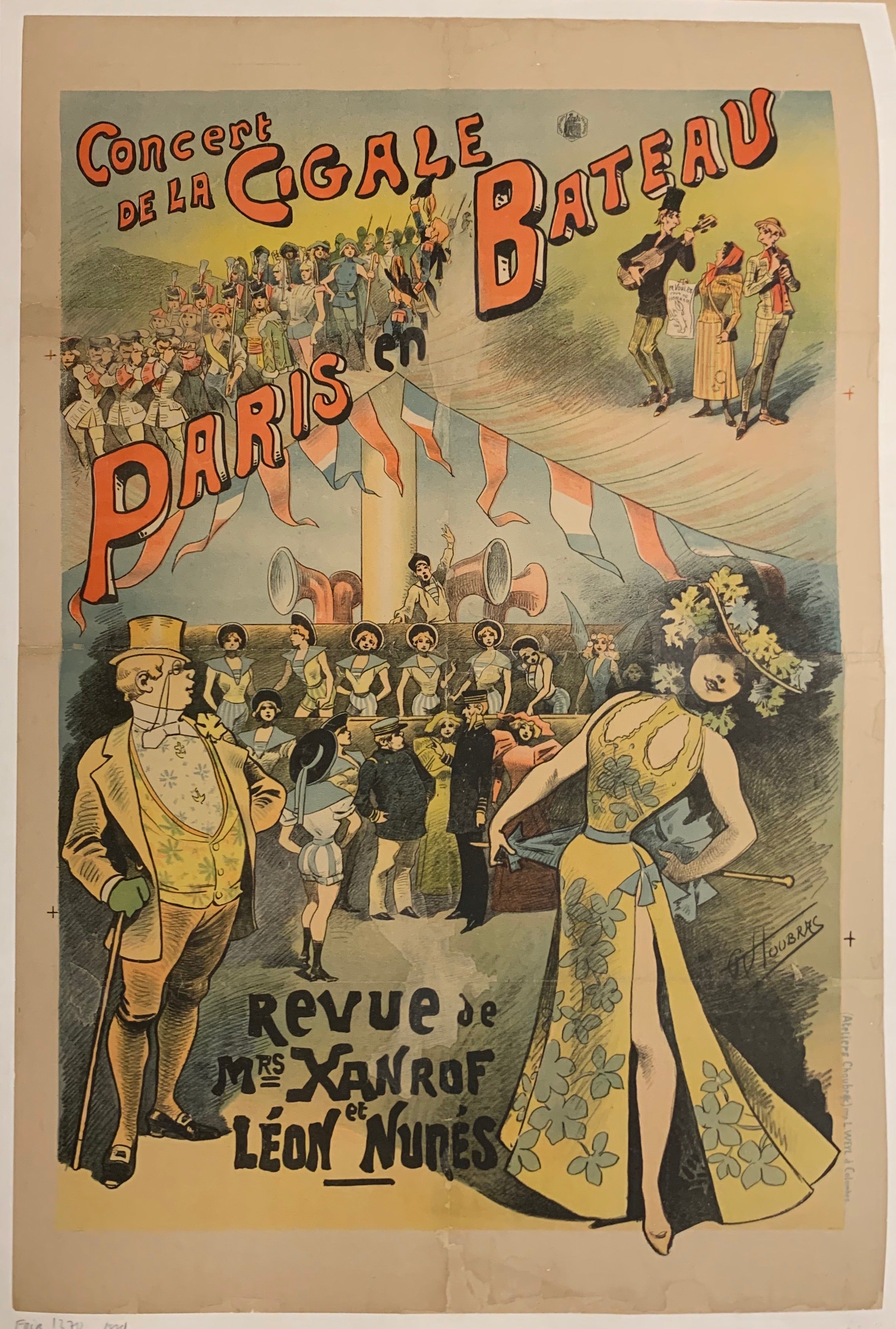This vibrant and detailed poster, seemingly from the early 20th century or earlier, advertises a Parisian event titled "Concert de la Cigali Bateau." The bright orange text at the top reads "Concert de la Seagalle 2," and below it, "Paris." Near the bottom, additional French text reads, "Review des Misses Zanroth et Leon Nunes," likely naming the event hosts. They are prominently illustrated in the foreground. The male host is dressed in a distinct yellow suit with a matching vest and golden hat, accessorized with green gloves, an eyepiece, short leggings, knee-high stockings, and black buckled shoes. To his right, the female host strikes a pose in a strapless yellow dress adorned with blue flowers, a blue belt, and a high slit revealing her left leg. She wears an elegant hat also embellished with blue and yellow flowers. The background features various performers and flags, suggesting a lively show with a possible circus or carnival theme, characterized by the colorful and flamboyant attire of all the characters.